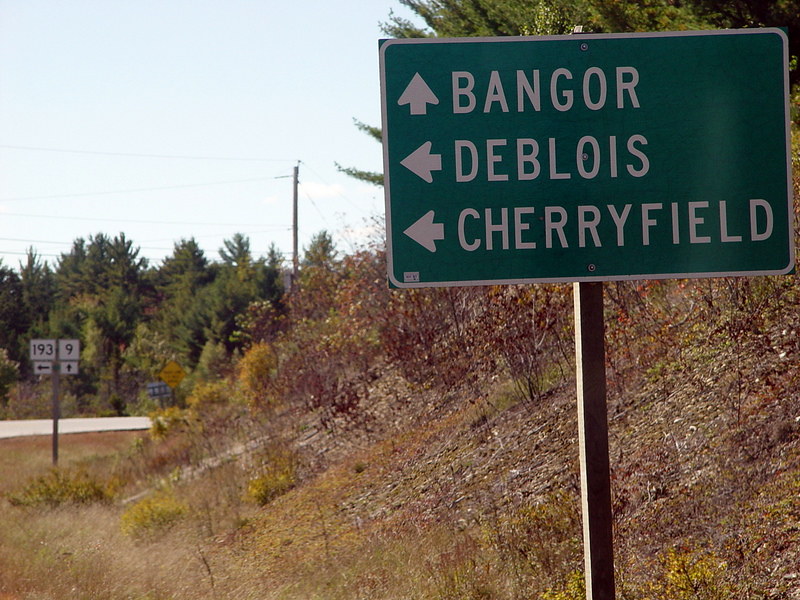In the outdoor photograph, the foreground is dominated by a patch of dry grass. On the far right side of the image stands a prominent green sign bordered in white. The sign features directional arrows with white text; the upper arrow points toward "Bangor," while the left arrows guide toward "Dublois" and "Cherryfield." A metal barrier arm, positioned at the bottom right, moves vertically. 

In the distance, the number "13" can be faintly discerned, and a forward-facing arrow points to "9." A gray road cuts through the scene, flanked by lush trees with green leaves that populate the background. Interspersed among the trees are utility wires and a pole, adding to the intricate landscape. The sky overhead is a muted gray, suggesting overcast conditions. At the bottom of the frame, a yellow sign punctuates the scene, adding a splash of color to the otherwise subdued palette.